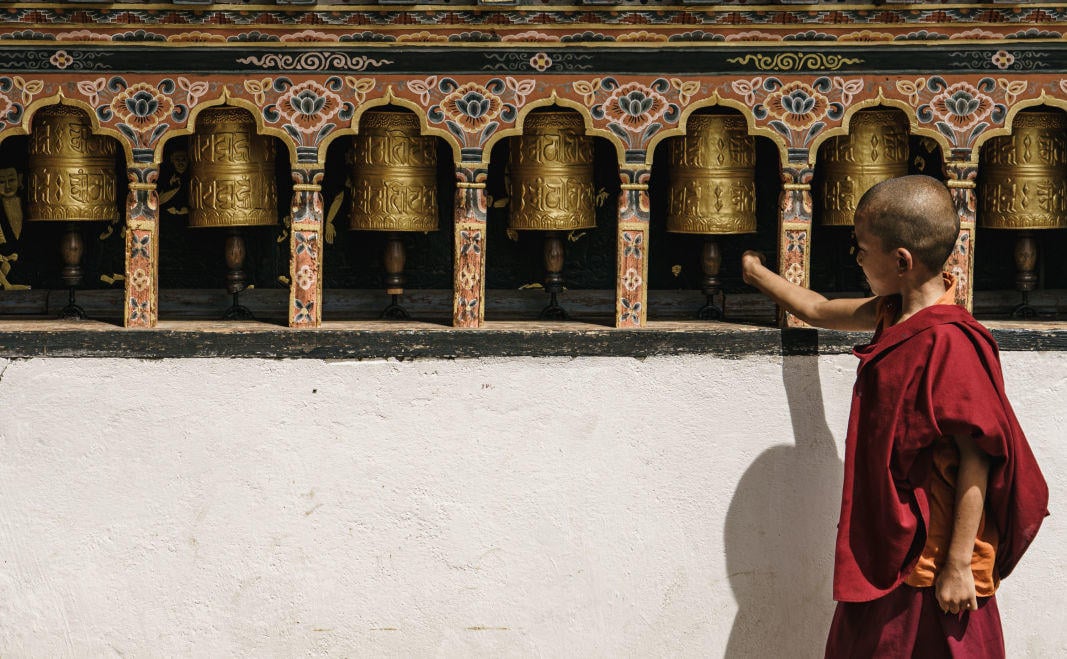In this image, a young bald boy resembling a Buddhist monk stands sideways, gently touching one of the seven ornate golden bells adorning a decorative wall. He is dressed in a dark red, drapey robe that wraps over his shoulder, complemented by an orange sash around his waist. The top part of the wall features intricate, multicolored designs in hues of red, brown, and blue, enhancing the serene atmosphere. Each bell, embellished with detailed designs, is housed within small, archway-like inlets. Below this, the wall transitions into a plain white surface. The golden bells boast intricate, embossed patterns, and their beauty is juxtaposed against the more subdued but equally exquisite designs on the wall.